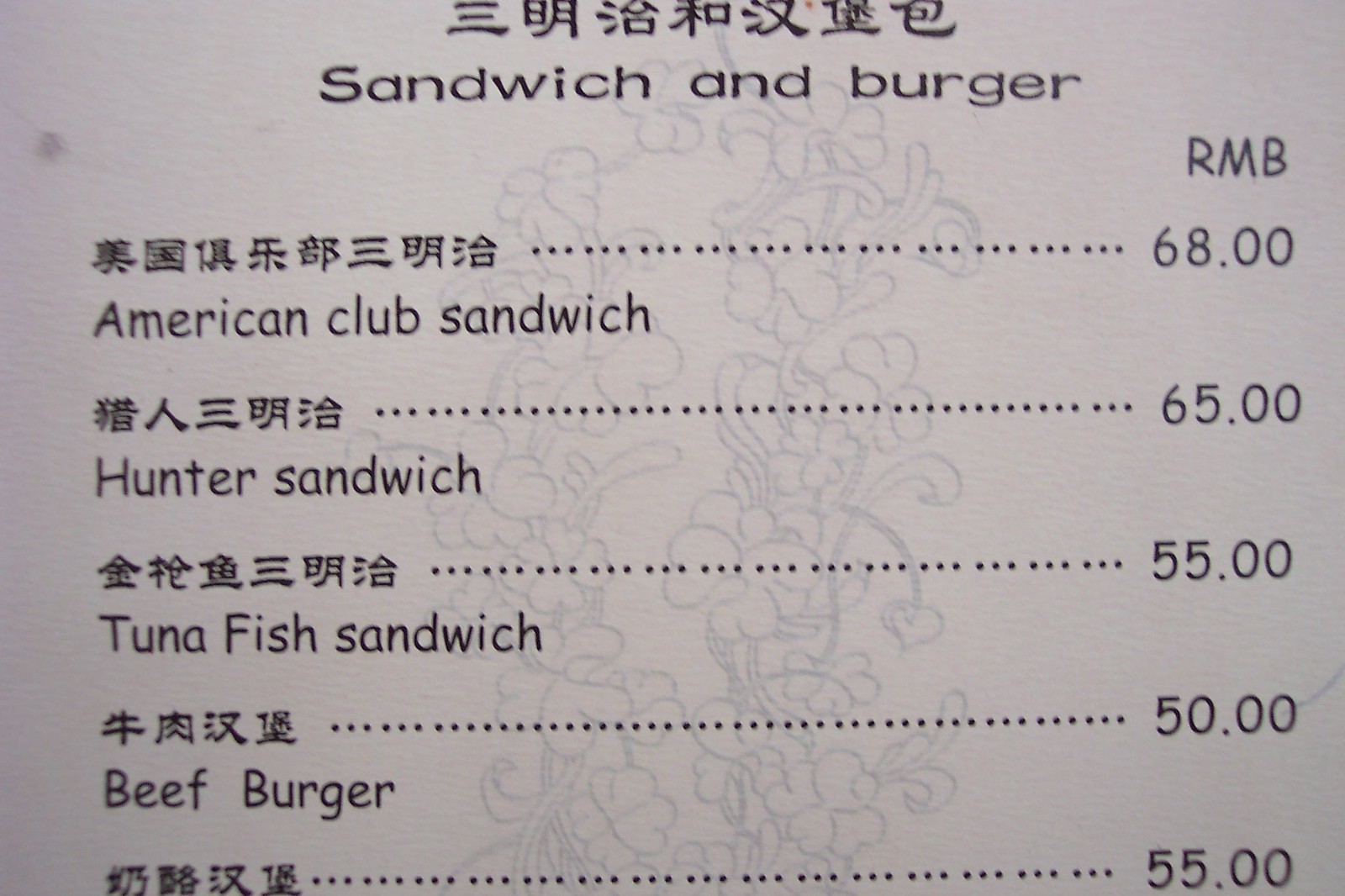This close-up image captures a bilingual menu featuring a selection of sandwiches and burgers. The menu is presented in black text on a white background, adorned with a subtle floral or herbal design. The Chinese characters above each item likely denote the names of the items in Mandarin. 

The menu items are as follows:
- **American Club Sandwich**: Priced at 68 RMB.
- **Hunter Sandwich**: Priced at 65 RMB.
- **Tuna Fish Sandwich**: Priced at 55 RMB.
- **Beef Burger**: Priced at 50 RMB.
- **Mystery Item**: Displayed only in Chinese characters, priced at 55 RMB.

This menu is possibly for a takeout restaurant, although the specific location is not visible in the image. The descriptive nature of the caption hints at choices being made: a tuna fish sandwich, a hunter sandwich, and a beef burger, suggesting personal preferences.